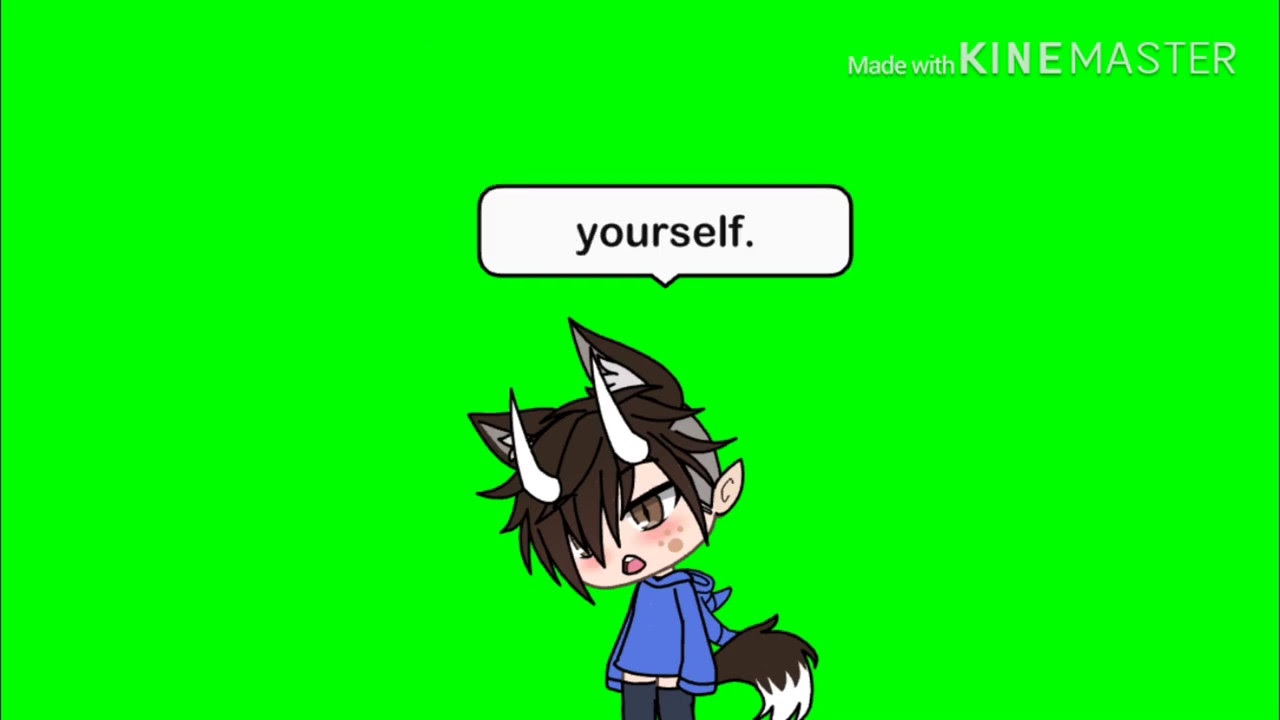The image features a detailed drawing of an animated cartoon character set against a bright green background. The character appears to be a little boy with a unique, whimsical appearance. He sports a blue long-sleeved shirt with a hood, blue pants, and black boots. His dark hair is complemented by two white horns protruding from his forehead and black pointy ears on top of his head, resembling fox or cat ears. He has a fleshy, white face with a paw print on his cheek, one large brown eye, and a partially hidden eye under his hair. A bushy, black and white (or brown and white) fox-like tail extends from his back. The character is facing forward with a slightly open mouth, appearing to engage the viewer.

In the background, there's a conversation bubble directly above the character's head, outlined in black with a tiny triangle pointing towards the character, indicating that he is speaking. Inside the bubble, the text reads "yourself." in lowercase black font. Additionally, in the upper right-hand corner of the image, the text "Made with KineMaster" is prominently displayed, with "Made with" written in mixed case and "KineMaster" in all uppercase letters.